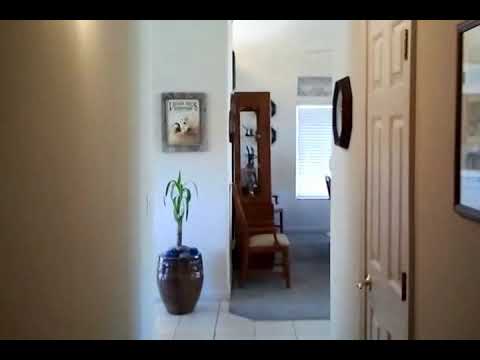This image captures a view through a doorway, looking from a hallway into what appears to be a dining room. The foreground of the photo is framed by a light brown wall on the left, which is blurry as if shot near a wall, and a beige wall on the right adorned with several pictures, a mirror with a dark wooden frame, and a white door with a brass handle and hinges. An octagonal clock with a dark wooden frame is also visible on the right wall. On the left side at the end of the hallway, a white wall with a mounted picture extends into the dining room. Below this on the lower left is a large brown pot holding a tall potted plant that looks like it could use some water. The hallway floor is tiled, transitioning to grey carpet in the dining room area. Inside the dining room, a window allows some light to filter in, creating white splotches of glare on the carpet and hinting at ceiling lights. There’s a brown curio cabinet decorated with various items, and to its left is a fancy chair, also with a brown frame. The image is presented with black horizontal bars at the top and bottom, indicating it might be a still from a piece of media.